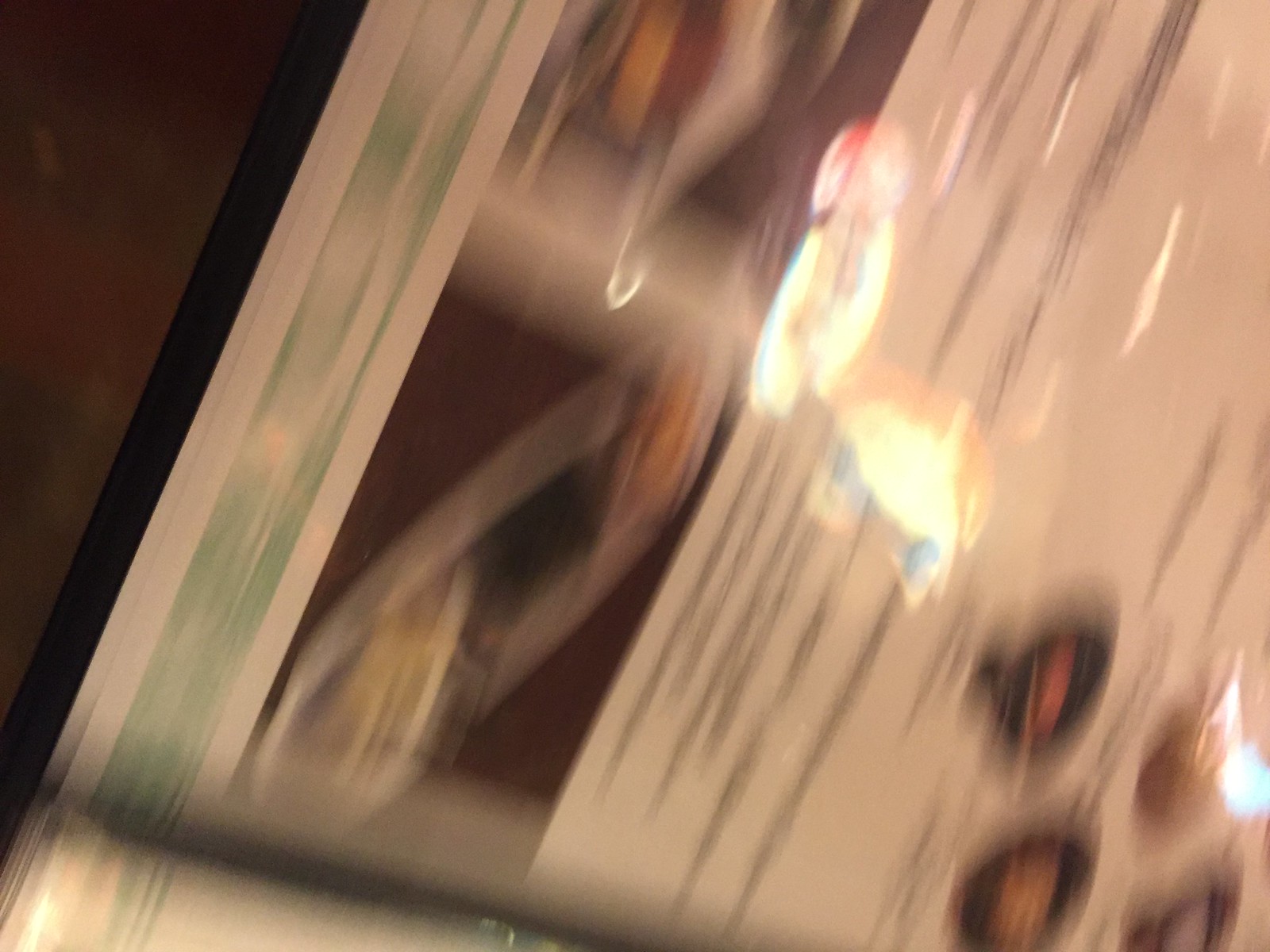This extremely blurry image features an indistinct subject that could be interpreted as either artwork or a glass object. The background, particularly in the top left corner, is a shade of brown. Diagonally traversing the image from the bottom right to the upper left is a black strip. Upon closer inspection, the image vaguely resembles the open page of a book, featuring highly blurred white pages. Reflected in the middle of the image are several overhead lights, emitting a bright, almost otherworldly white glow. Paralleling the black line on the right side is a green strip. Overall, the scene is dominated by an interplay of gray and white hues, punctuated by black circular elements.